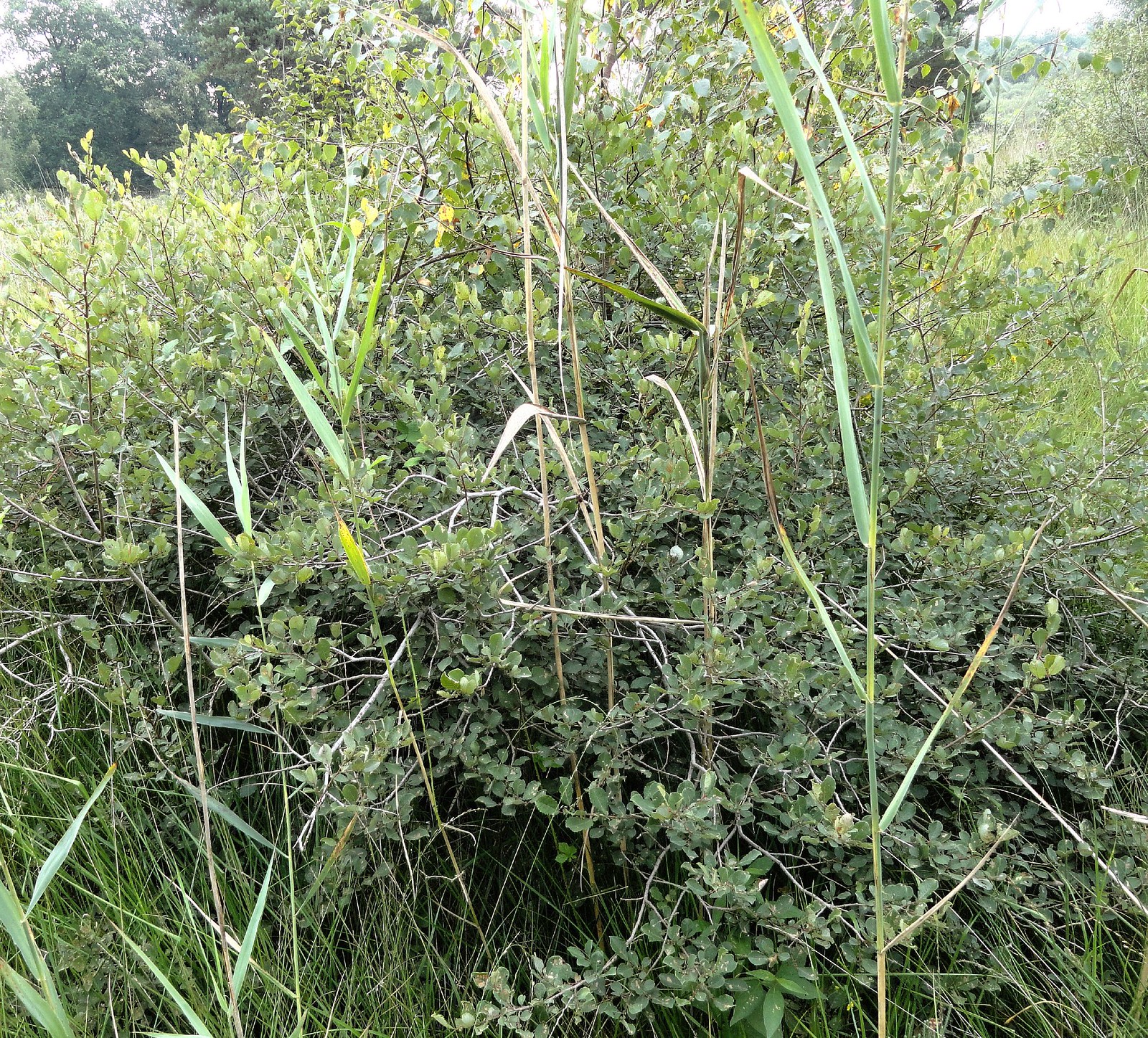This is an outdoor, daytime photo capturing a lush, green scene in what appears to be a forest. The square image focuses closely on a dense area of greenery dominated by bushes and tall grass, with various plants and wildlife interspersed. The predominant foliage includes medium-height bushes with numerous small green leaves and some with lighter, almost yellow leaves. A noticeable tall stalk of wild grass rises prominently in the foreground. Sunlight filters through the scene, particularly illuminating the left side. The sky is only slightly visible, appearing white in the upper left and upper right corners. In the background, there are hints of dark green trees, providing a subtle contrast to the vibrant, sprawling greenery in the forefront.